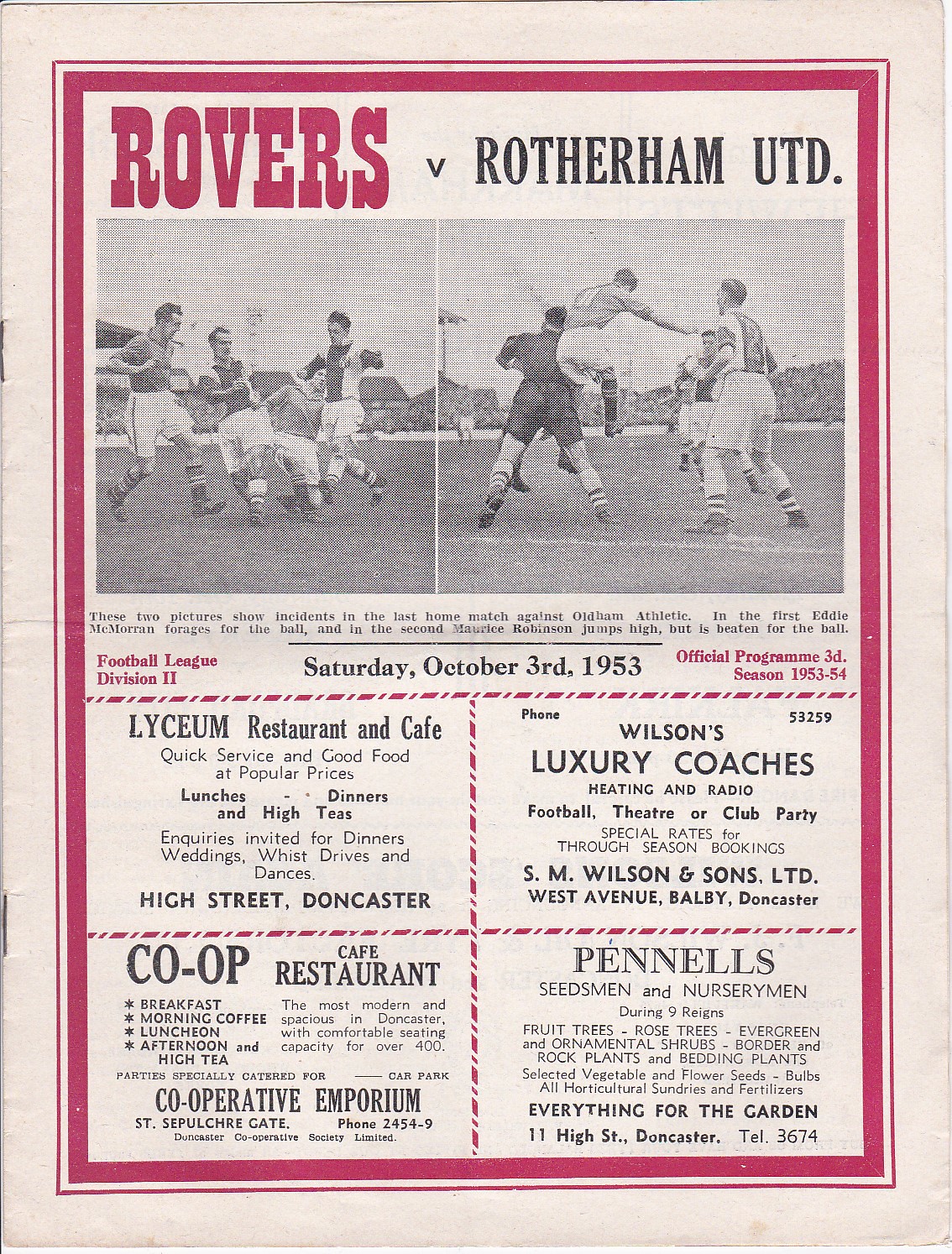This is a vertically oriented rectangular scan or photograph of an old football program cover, fastened with two staples along the left side. The cover, appearing off-white and slightly weathered, features a thick red border. Dominating the top half of the cover, the title "ROVERS" is printed in large red letters, while "V ROTHERHAM UTD" appears in black letters beneath it. Below the titles are two prominent black and white photographs depicting football players in action: on the left, three players contest for the ball, and on the right, one player leaps into the air as two others look on. Directly beneath these photos, text announces "Football League Division II, Saturday, October 3rd, 1953, Official program season 1953-54." The bottom portion of the cover displays a two-by-two grid of advertisements separated by dashed red lines. The advertisements are for Lyceum Restaurant & Cafe, Wilson's Luxury Coaches, Co-op Cafe Restaurant, and Pennell's Seedsmen and Nurserymen.